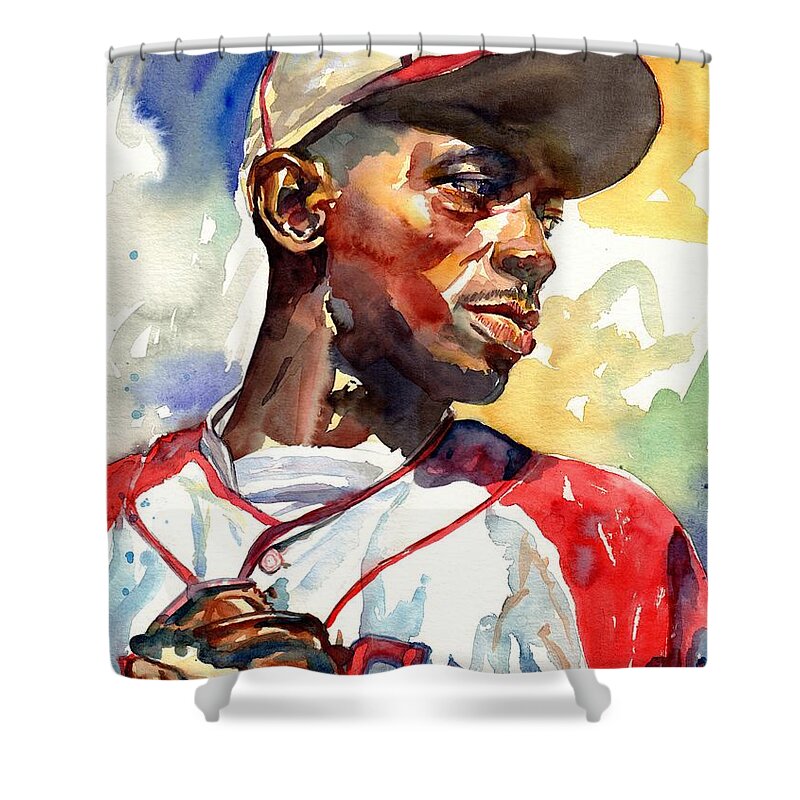This image depicts an artistic shower curtain adorned with a vivid watercolor and oil canvas-style painting of an African-American baseball player. The player, characterized by his black complexion and thin mustache, dons a striking red and white jersey with a white undershirt, and a cap, and his posture reveals a relaxed yet focused demeanor as he gazes over his left shoulder. His torso faces forward while a brown glove is visible near the bottom left corner of the curtain. The background is an abstract blend of blues, greens, yellows, and whites, creating a lively and textured effect. The curtain hangs from a white horizontal shower rod with rings, revealing the feet and base of a claw-foot bathtub below, situated against a clean, white backdrop. This meticulous representation merges the essence of sports with a splash of contemporary art.